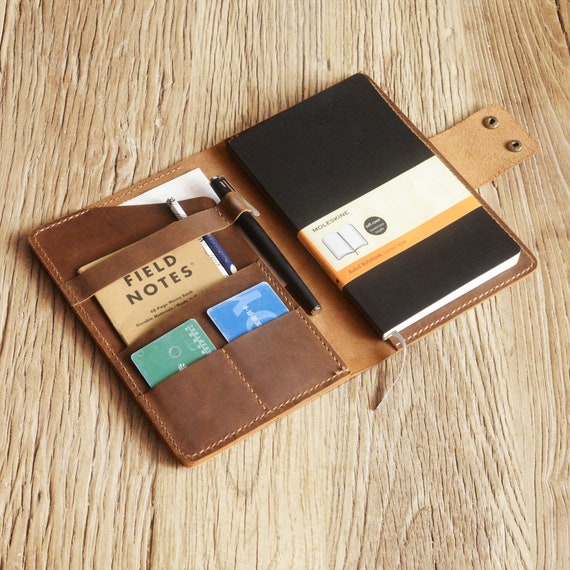The image shows an open, almost leather-like tan binder laying flat on a light woodgrain table. On the right-hand side, there is a brand-new, wrapped Moleskine ruled notebook complete with a cloth bookmark. The notebook is securely hooked inside the binder using the bottom flap. Adjacent to the notebook, there's a holder containing a black ink pen. On the left-hand side of the binder, there are multiple sections: a large pocket for papers, a smaller pocket holding a booklet labeled "Field Notes," and two smaller slots containing credit cards—one blue and one green. Additionally, a second ink pen, blue and white, is visible. The binder, designed with two snaps for closure, effectively organizes and carries various essentials such as the notebook, writing instruments, and credit cards.